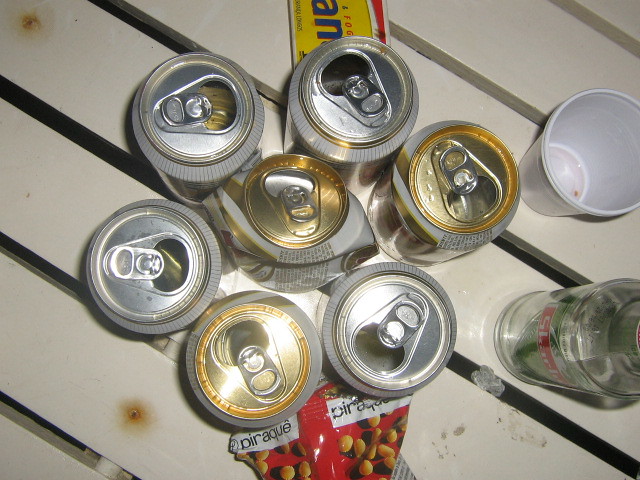The image depicts a white outdoor table made of wooden slats, viewed from above. Arranged on the table are eight predominantly opened beer cans, seven of which form an uneven circle with one crushed can in the center. Additional details include an eighth can positioned off to the side. Nearby, a white plastic cup and a small glass bottle with a red tag are visible. The bottom of the image shows a snack bar wrapper, with the brand "Para-Q" marked by a distinctive upward-pointing arrow over the "E". The wrapper appears to be non-English and could possibly depict candy or nuts. At the top of the image, partially obscured by a beer can, is another wrapper colored yellow, red, and white. The nails securing the table's slats exhibit some rust, adding a touch of weathered character to the scene.